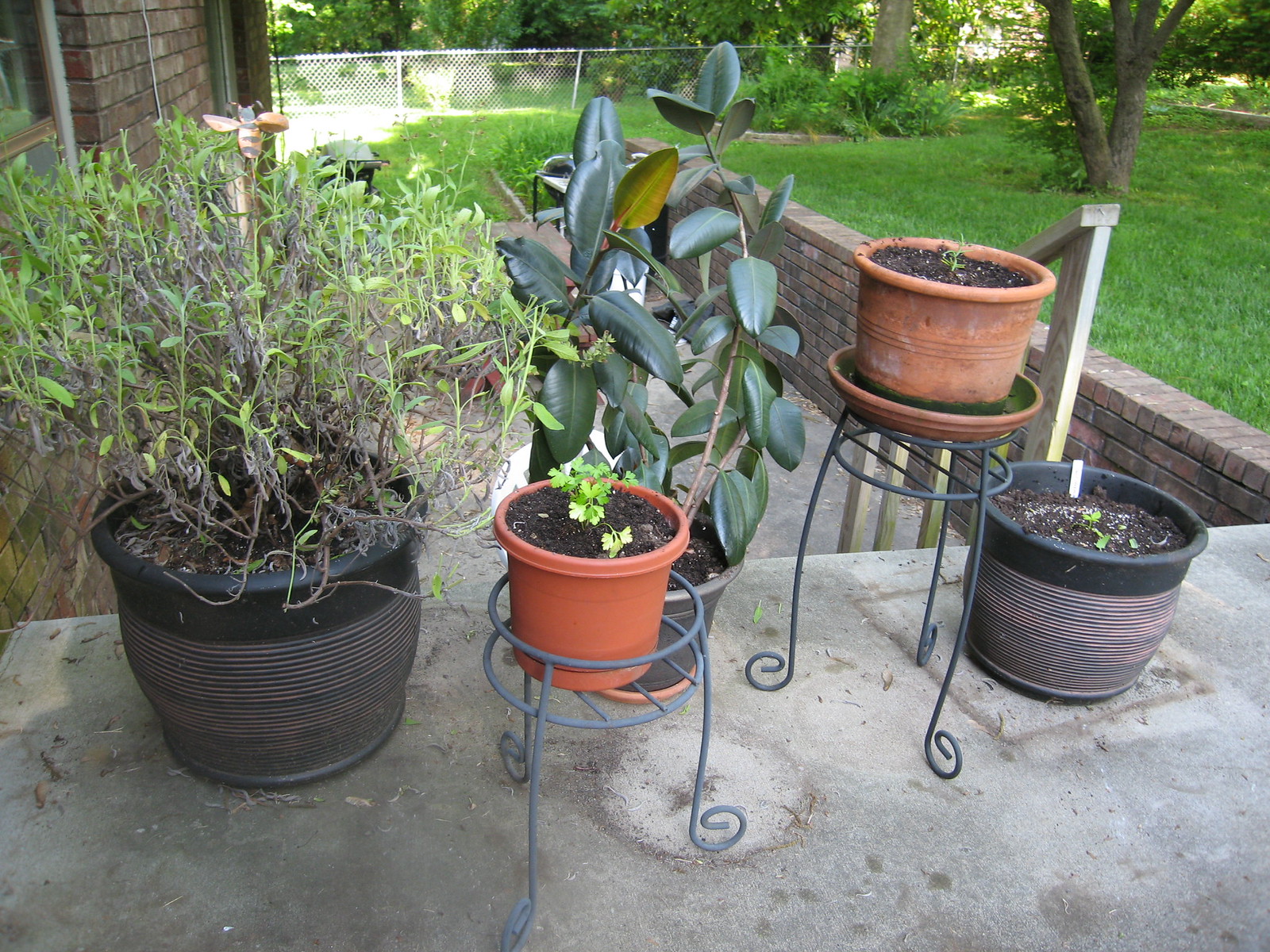This image captures a tranquil outdoor area adjacent to a brick house, featuring a well-arranged collection of potted plants on a cement patio. There are five distinct pots, each with unique greenery. On the left, a black pot with brown stripes houses a slender shrub with numerous upward-pointing green leaves, adorned by a decorative bee stake. Centrally located, a large ficus with lush, dark green leaves sits in a black pot, trimmed by a smaller terracotta-colored plastic pot on a black metal stand, likely containing parsley or cilantro. To the right, another black metal stand cradles a terracotta pot and saucer with a very small green plant sprouting. Adjacent to this stand, a similar black striped pot on the ground holds fledgling green plants. The scene is complemented by a backdrop of a grassy yard, a tree line, and a chain-link fence, with a brick wall partially visible on the left, suggesting the composition is part of a serene backyard retreat.